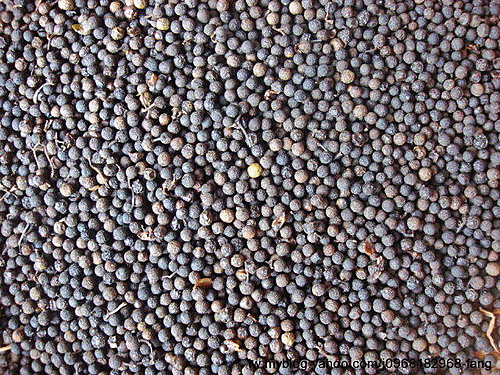This close-up aerial photograph showcases a densely packed assortment of small rocks, marbles, or gravel scattered over the ground. The scene is devoid of any specific focal points such as people, animals, or prominent objects. Thousands of these varied objects fill the frame, creating a textured and colorful mosaic. Predominant colors include light blue and gray, interspersed with white, black, and the occasional red-tinted stone. The uniform yet varied arrangement resembles a natural cluster or a deliberate spread, with the daylight highlighting the different tones and details, reminiscent of a field of blueberries or an expanse of peppercorns. Each object appears to be randomly placed, some chipped or cracked, revealing lighter interiors, adding to the intricate visual tapestry.